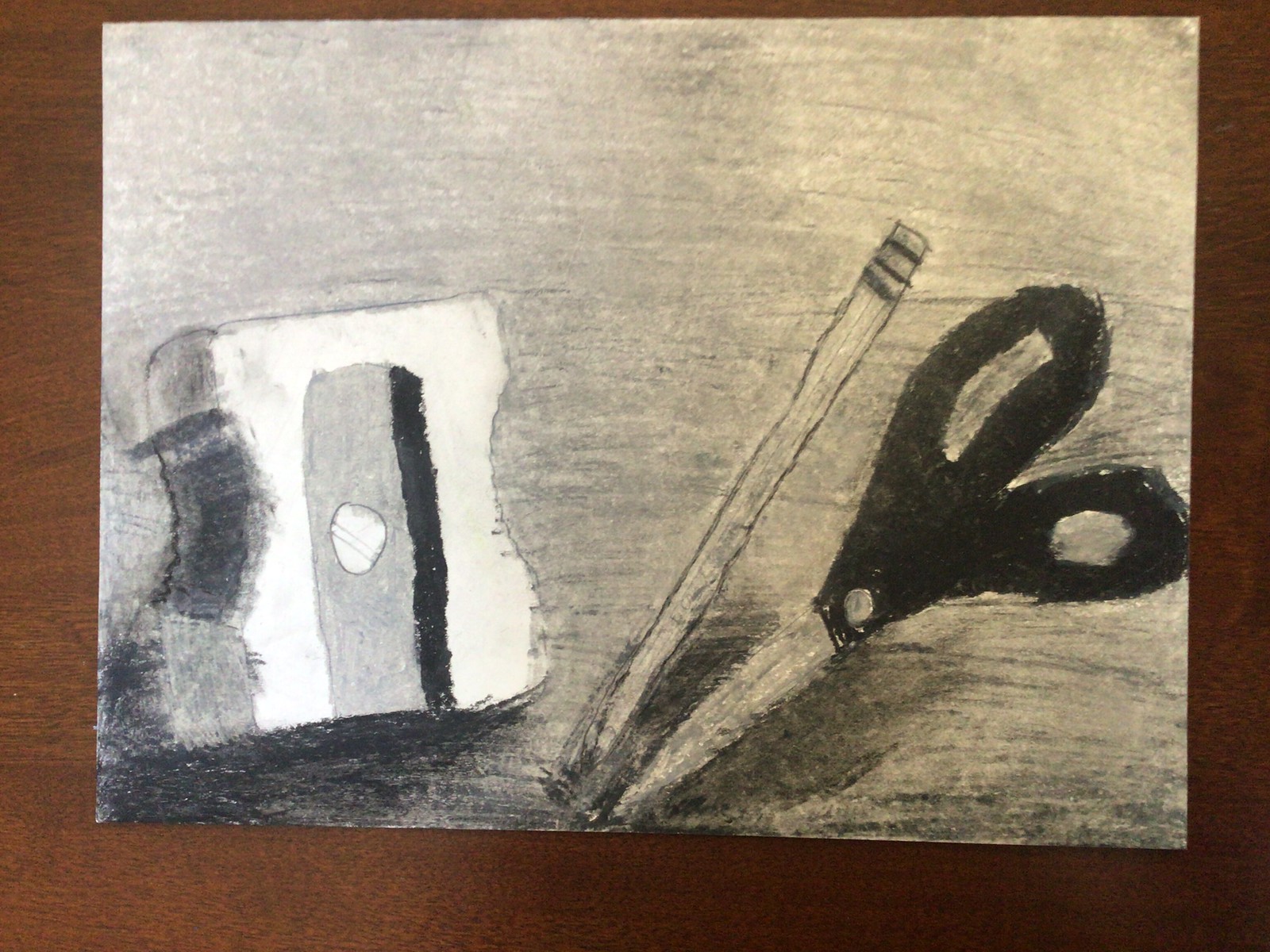The image depicts a detailed charcoal drawing on a white rectangular piece of paper, set against a dark brown wood grain tabletop. The paper, entirely shaded in a light gray tone, features several distinct objects. On the left side, there is a meticulously drawn square-shaped notebook or possibly a hand pencil sharpener, characterized by a shaded line down its center and a small screw-like detail. Directly to its right is a pencil angled upwards towards the right corner of the page. Below this pencil, a pair of scissors with dark black handles sits prominently, with their pointed tips directed downward. The shading is darker towards the edges, adding depth and contrast to the composition.